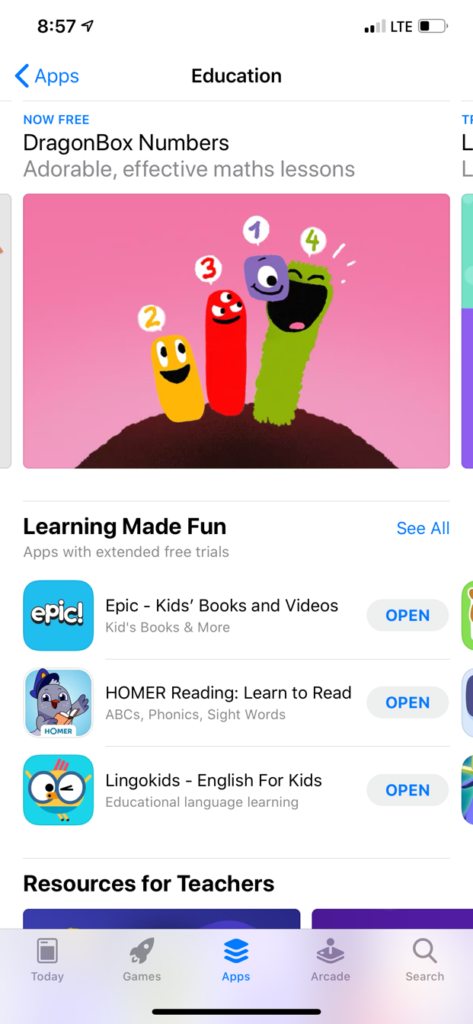Screenshot of an education-focused mobile app interface, captured at 8:57 AM. The top status indicators show a cell signal strength of 2 out of 4 bars, LTE connectivity, and a battery level at roughly one-third full. 

The main content area highlights "DragonBox Numbers," a free and engaging math app featuring lessons with adorable characters. The screenshot prominently displays four cartoon worms, each numbered and color-coded: worm 1 is purple, worm 2 is yellow, worm 3 is red, and worm 4 is green, making learning fun and interactive. 

Below this, there's a section titled "Apps with Extended Free Trials" showcasing several educational apps. These include:

- **Epic!**: "Kids Books and Videos," with an option to open.
- **Homer Reading**: "Learn to Read, ABCs, Phonics, Sight Words," with an option to open.
- **Lingokids**: "English for Kids, Educational Language Learning," with an option to open.

At the bottom, a bold header reads "Resources for Teachers," accompanied by icons for "Today," "Games," "Apps," "Arcade," and a search icon. There are visual cues suggesting more content available via lateral swiping, hinting at additional resources just out of the current view frame.